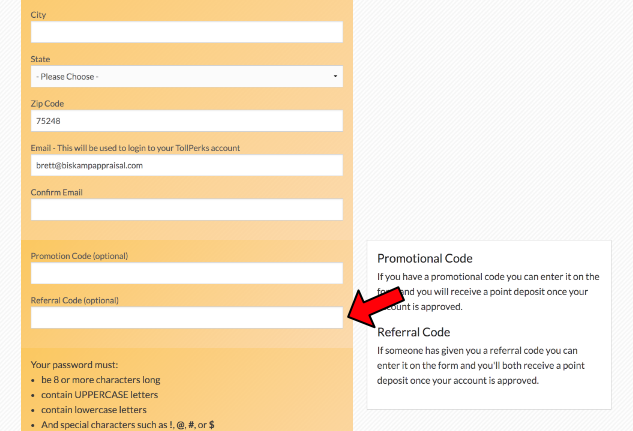The image displays a user registration form for a rewards program, vividly designed with gold outlines. 

At the top of the form, the word "City" appears in black text followed by a white input field where users can type in their city. Below this, the label "State" is also in black text, paired with a white selection banner labeled "Please choose," which prompts a dropdown menu for users to select their state.

Next is the "Zip Code" field with an adjacent white box for typing in the zip code. Following it, the form asks for an email address with the note, "This will be used to log in to your toll perks account." An example email, "brett@briskampraisol.com," is filled into a white input field.

Immediately below, users are prompted to confirm their email address by retyping it into another white input field. Then, the form provides fields for an "Optional" promotional code and referral code, each accompanied by a white input box.

Towards the bottom of the form, instructions stipulate that the user’s password must:
- Be eight or more characters long
- Contain uppercase letters
- Contain lowercase letters
- Include special characters such as !, @, #, or $

Next to the referral code field, a banner has popped up on the right side with the following text in black: 
"Promotional Code: If you have a promotional code, you can enter it on the form and you will receive a point deposit once your account is approved.
Referral Code: If someone has given you a referral code, you can enter it on the form and you'll both receive a point deposit when your account is approved."

This banner is highlighted with a large red arrow pointing towards the referral code field, and the arrow is outlined in black for emphasis.